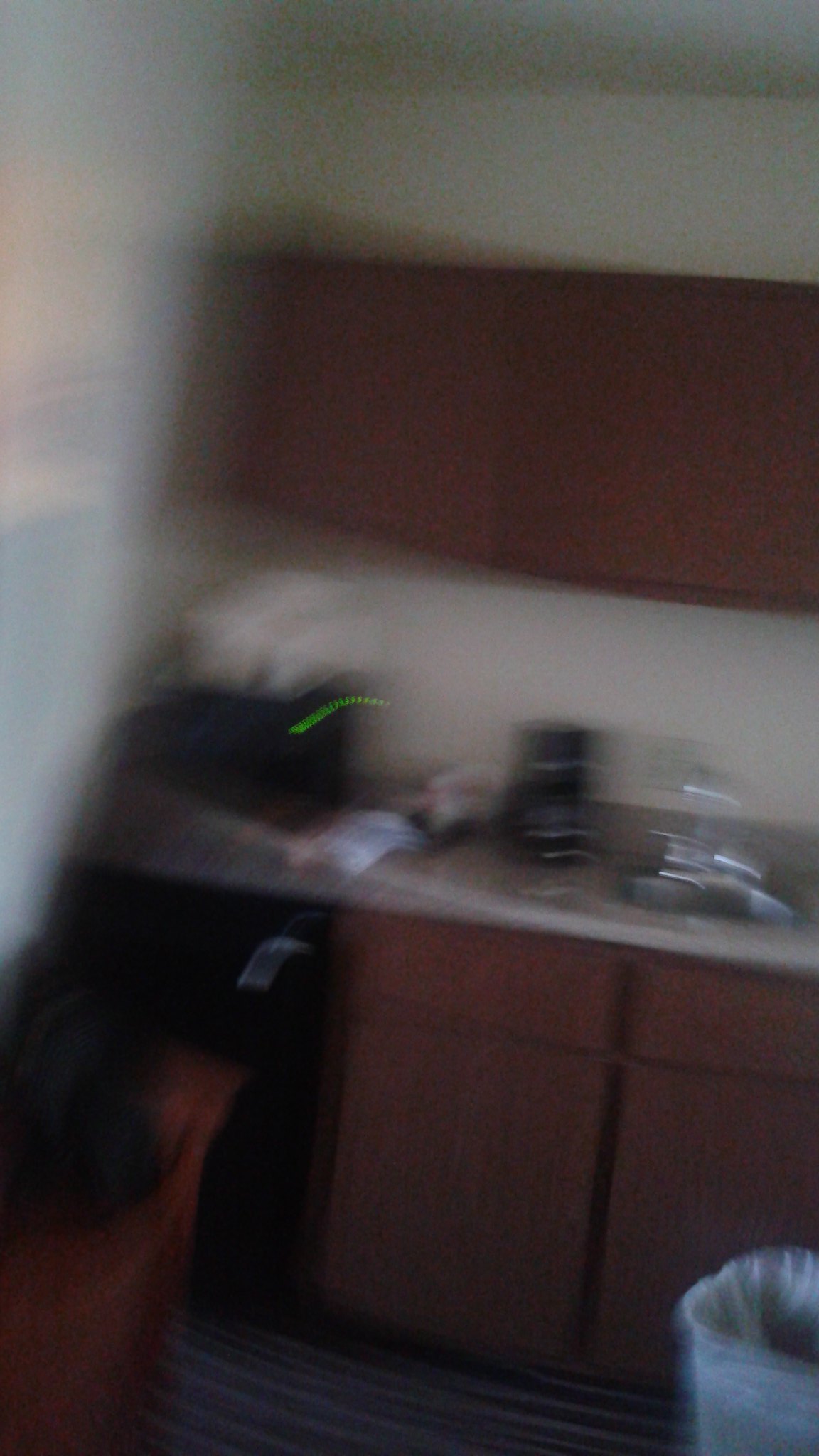A very blurry indoor photograph captures a segment of a kitchen space. The image includes an off-white wall with brown wooden cupboards mounted above a counter made of a gray, marble-like material. On the right side of the countertop, a chrome sink with a matching chrome faucet is partially visible, though distinctly out of focus. Positioned to the left of the sink sits a small automatic coffee maker. Adjacent to this coffee maker, there are two small, white packages resting on the countertop. Further to the left, there appears to be a microwave oven, above which a black shape featuring a fuzzy green smear likely represents a digital clock display. In the lower right corner of the image, a wastebasket is discernible.